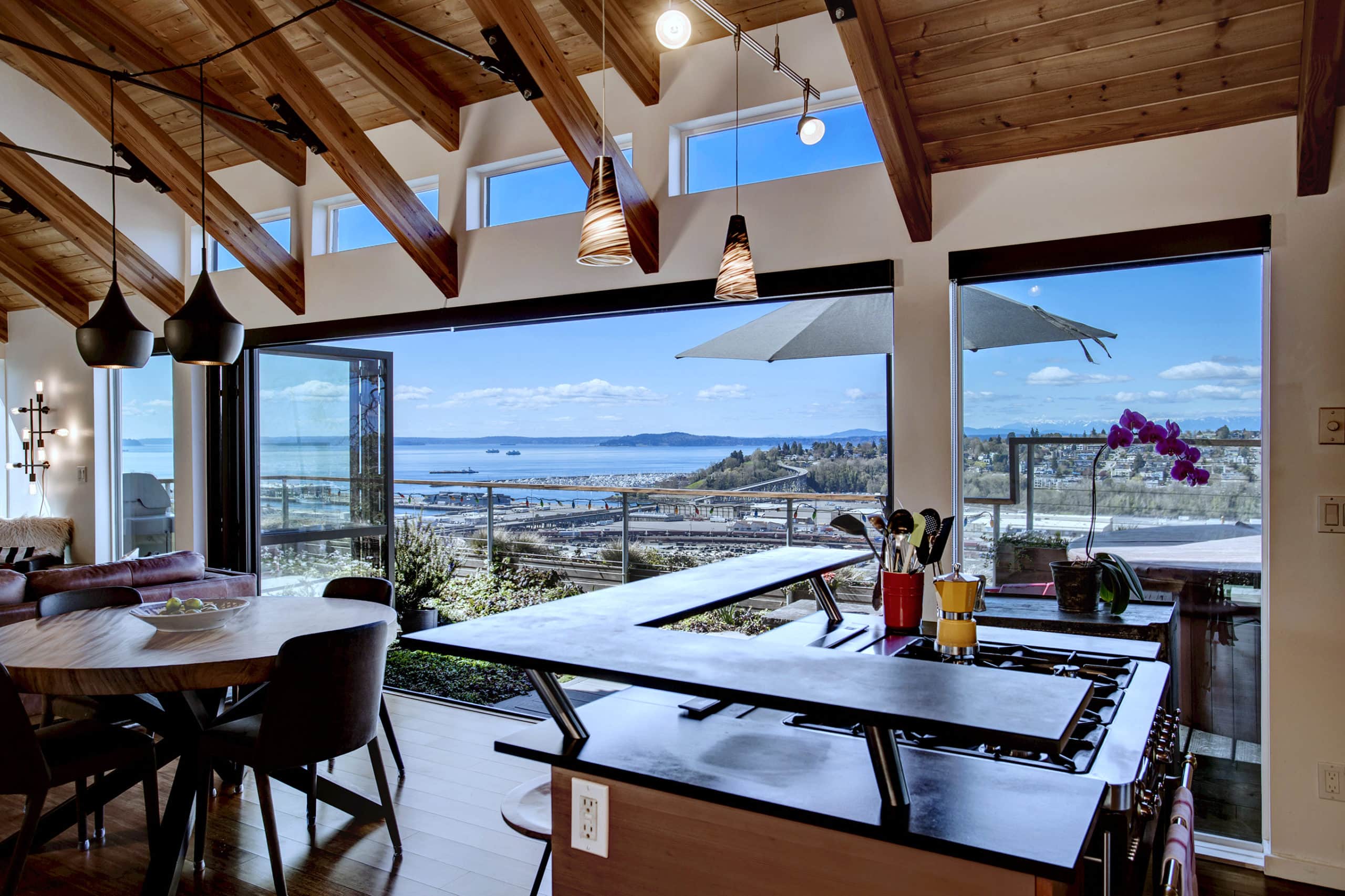This color photograph showcases a modern kitchen and dining area with minimalistic decor. In the foreground, a black gas cooktop with controls on the right-hand side sits on a wooden base, with a counter nearby holding various utensils, including a coffee pot and a large red glass container. To the left, a round wooden dining table with four black chairs has a bowl of fruit as a centerpiece. The room's white walls feature a wall sconce and a beam that runs across the ceiling, which is adorned with cone-shaped, hanging accent lights. The kitchen and dining area is illuminated by natural light streaming in through a large picture window and additional windows to the right, with a door on the left leading to a patio with green plants and a railing. Beyond the patio, the expansive landscape includes a body of water to the left, a distant mountain range, and a tree-covered hill with houses to the right. A roadway can also be seen winding up the hill, with the scene completed by a dock and a small city visible outside under blue skies with a few scattered clouds.